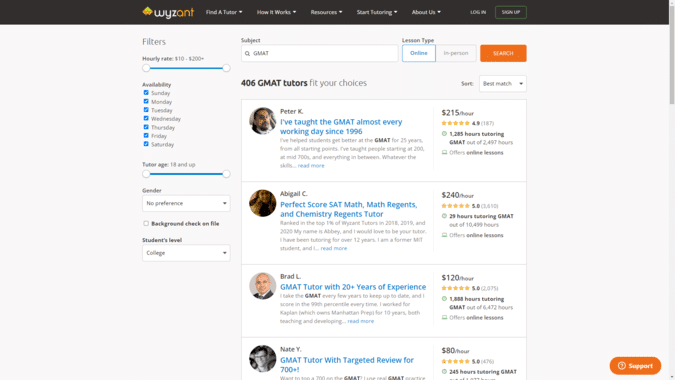This horizontal, left-to-right image depicts a website interface that appears to be designed for both desktop and smart device access. The background is a flat, medium to light gray with no texture or dimension. 

At the top of the page, there's a black rectangular strip with the "Wyzant" logo situated on the upper left. Next to the logo, there are several navigation options: "Find a Tutor," "How it Works," "Resources," "Start Tutoring," and "About Us." Towards the right side of the strip, there are "Log In" and "Sign Up" buttons, with the "Sign Up" button highlighted by a green box.

On the left of the screen, there are various filters for refining search results: hourly rate ranging from $10 to $200+, availability with all days checked (indicated by blue boxes around checkmarks), tutor age (18 and up), gender (with "No Preference" checked), and background check status (currently unchecked). The student level filter is set to "College," but is customizable.

At the top center, the subject field indicates "GMAT," and the lesson type is set to "Online" (though in-person is also an option). The search indicates there are 406 GMAT tutors available that fit the selected criteria. The results can be sorted by "Best Match." Each tutor listing includes their name, a brief description, hourly rate, star ratings, and reviews.

Overall, the image provides a detailed look at the functionality and layout of the Wyzant tutor search interface.